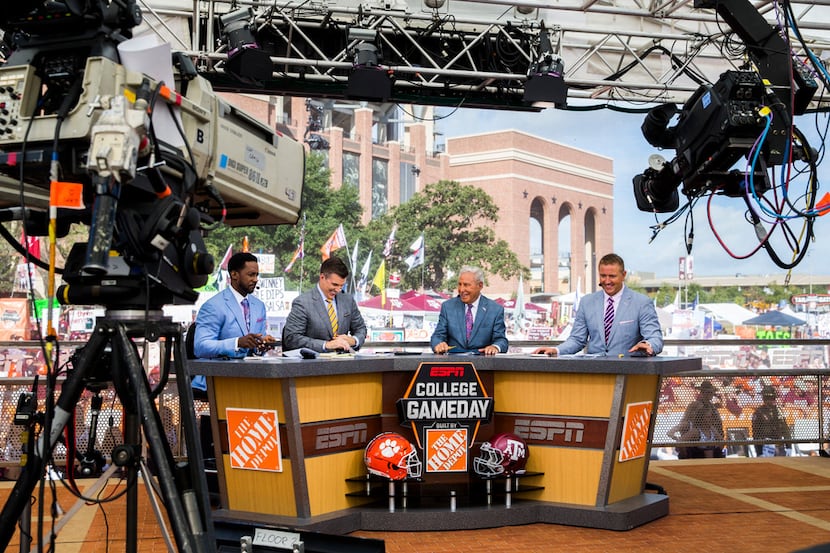Behind the scenes on the ESPN College Game Day set, four men in elegant suits—a black man with a purple-blue tie, and three white men—are engaged in conversation at a meticulously arranged L-shaped desk. The gentlemen sport a variety of suit colors, mainly blue and one gray, each complemented by distinctively colored ties: yellow, purple, and striped pink and black. Dominating the center of the desk is a sign that reads "ESPN College Game Day," flanked by the Home Depot logo and decorated with football helmets from the Clemson Tigers and Texas A&M Aggies. The backdrop is vibrant with a bustling crowd, flags, tents, and a large university building, indicating an ongoing college tailgate party. Above the set, an elaborate network of crisscrossed wires and lighting rigs, alongside multiple focused cameras, creates an atmosphere of organized chaos. The scene captures the anticipation and excitement of the upcoming football game while the hosts, deep in discussion and shared laughter, add a lively touch to the professional studio setup.